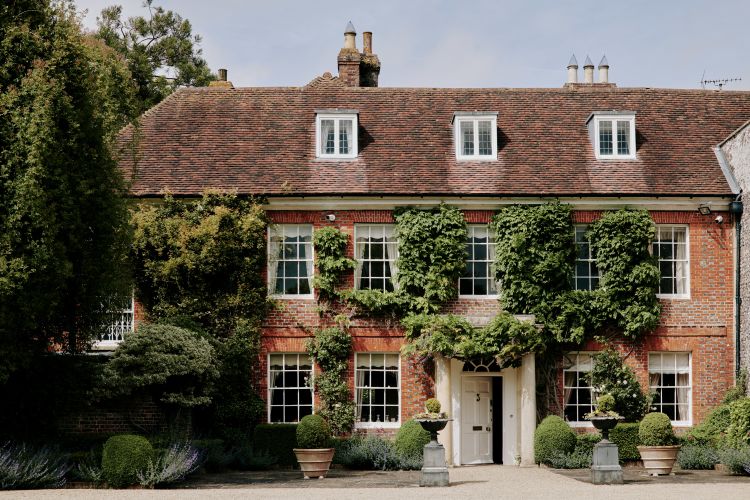The image depicts a large two-story brick mansion with a brown roof, featuring several chimneys and intricate architectural details, including pointy roof elements. The facade of the house boasts nine windows: four on the lower story and five on the upper story, all adorned with white window panes. Additionally, three attic windows peek out from the roof, hinting at an expansive upper level. A white front door, slightly ajar, stands at the center, inviting yet mysterious. Surrounding the house is a lush array of greenery, including a mix of potted plants and naturally rooted flora. Trees flank the left side of the house, contributing to the picturesque, clear daytime setting. The photo captures the essence of a serene, well-maintained, and grandiose residence.